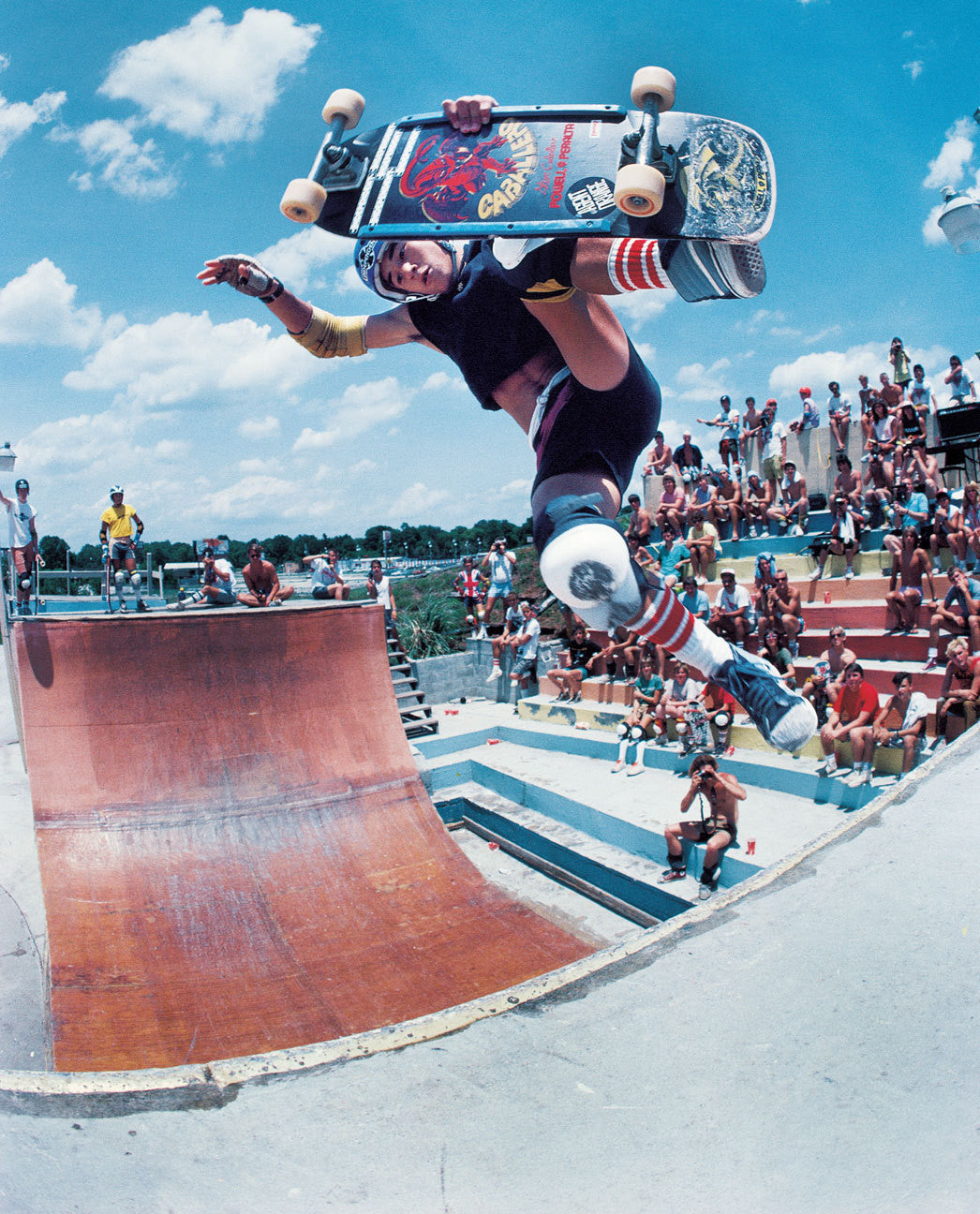The photograph captures a vintage scene of a skateboarder performing a mid-air flip trick on a wooden skate ramp, set against a clear blue sky with a few clouds and green trees in the background. The skateboarder is facing forward with his right leg down and his left leg up, holding the skateboard with one hand while his right arm is extended. He is dressed in an extremely tight black shirt and shorts, white knee pads, yellow elbow pads, tall white socks with red stripes, black shoes with white bottoms, and a black helmet. The skateboard has white reels and features a logo that includes the text "Kabbaler" and images of a red devil and a strange dragon-scorpion creature, along with various stickers. Below him, on the red skate ramp, a crowd of spectators in various clothing watches intently from an auditorium-like section with steps. In front of the crowd, a person with a small camera captures the action.